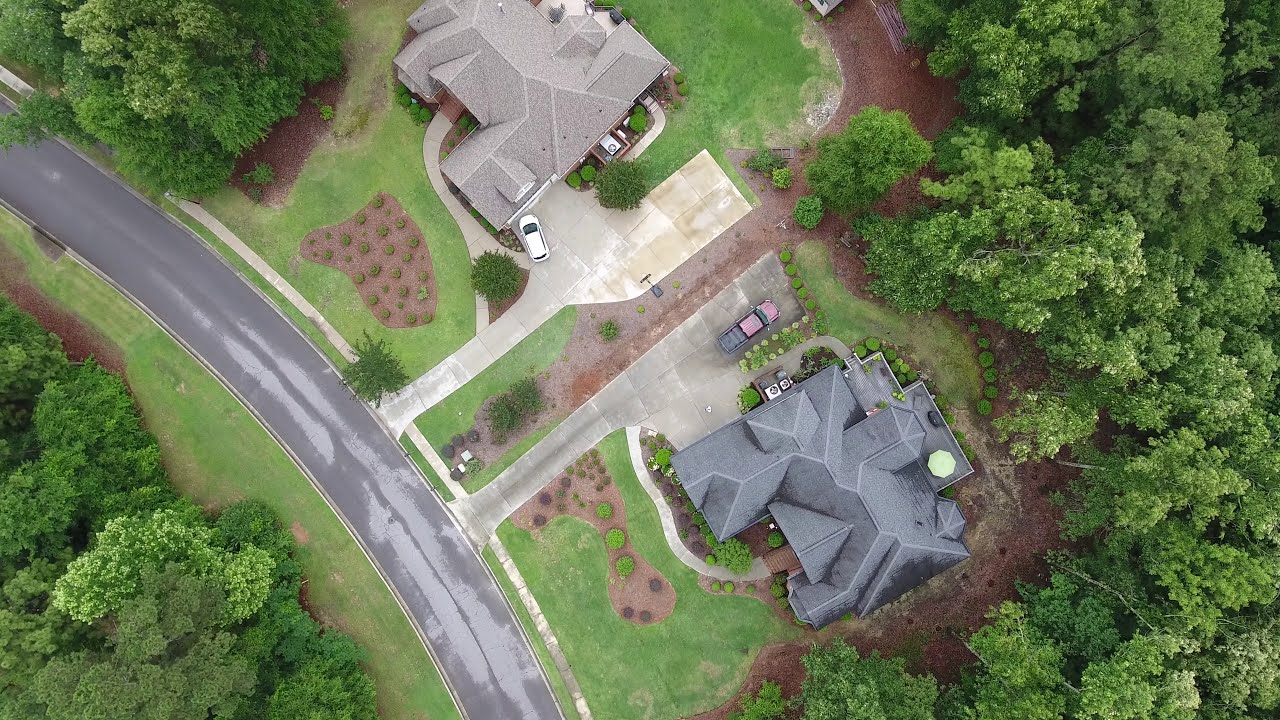This detailed overhead photograph, presumably captured by a drone or from an airplane, showcases two expansive McMansion-style homes in a rural setting. The home positioned in the bottom right corner features a darker gray, multi-segmented roof with various geometric shapes such as triangles and octagons. It is complemented by a large concrete driveway with a car parked in front and a pathway leading up to its front door, flanked by green bushes. Surrounding this home is a lush green lawn, extending both in front and behind, with a dense wooded area to the right.

The second home, located in the top left portion of the image, displays a lighter gray roof with similarly intricate segments. Its driveway, also gray and substantial in size, has a white car parked near the house. This home is surrounded by green lawns and additional bushes. There is a narrow strip of land separating the two properties.

A gray paved roadway arches from the top left edge of the image to the bottom, connecting directly to the driveways of both homes. This road, alongside the lush vegetation including patches of green grass and various groves of trees in the top left and bottom left corners, frames the entire scene with vibrant greenery, presenting a tranquil and picturesque rural environment.